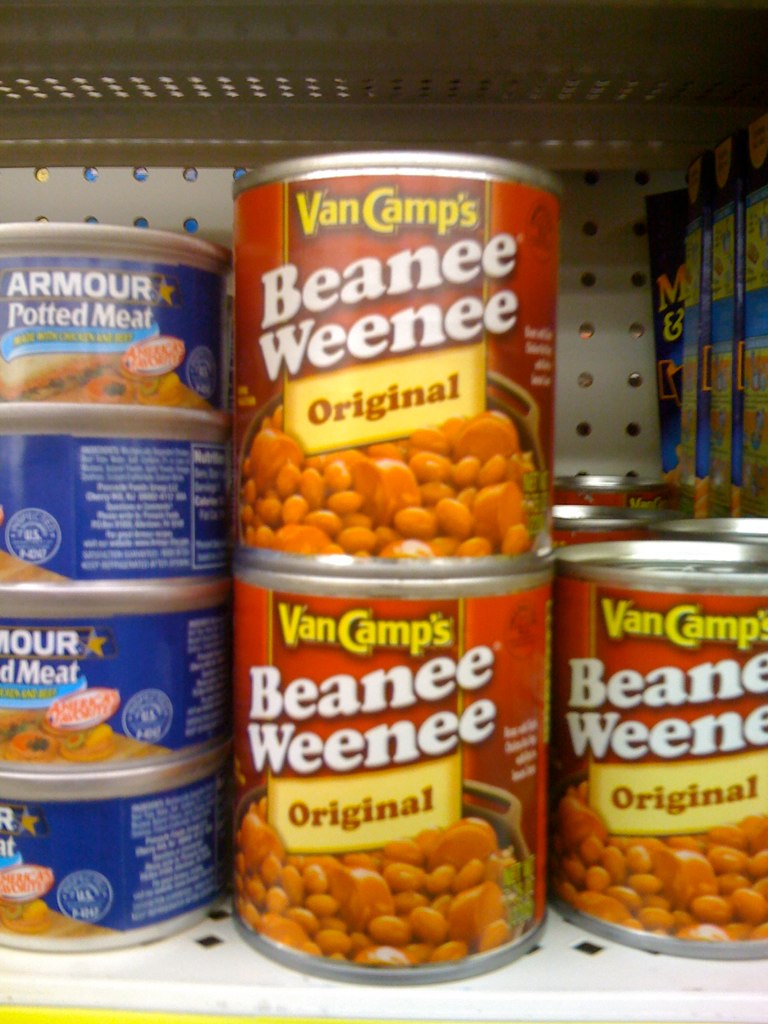In this full-color photograph, we see a market shelf stocked with cans. On the right side of the image, there are three cans of Van Camp's Beanee Weenee Original, a combination of beans and franks. These cans feature a vibrant red label, prominently displaying an image of a bowl filled with baked beans and slices of hot dogs. To the left, there are four blue cans of Armour Potted Meat, stacked one on top of the other. The label clearly reads "Armour Potted Meat". The shelving unit is typical of a market setup, made of white metal with slots and openings. Some of these openings are circular, while others on the bottom shelf are diamond-shaped, providing ventilation and stability for the cans.